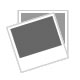The image is an advertisement showcasing a rugged, camouflage-decorated, all-terrain vehicle (ATV) known as the "Good Protector." The ATV, primarily black with khaki and camouflage elements, is depicted half-submerged in a river and emerging onto a rocky gravel path. Two people, dressed in black with helmets on, occupy the front seats of the vehicle. The image emphasizes the ATV's durability, focusing on a protective guard designed to shield the undercarriage, rear suspension, and taillights from rough terrain. A red line in the image highlights this protective feature, connecting to a close-up inset of the guard. The background features an autumnal landscape with a riverbank lined with rocks and trees, distant snow-capped mountains, and a partly cloudy blue sky. The text in the image reads, "Good Protector - protects the undercarriage, rear suspension, and taillights from being hit on tough terrain," underscoring the ATV's resilience and suitability for challenging conditions.